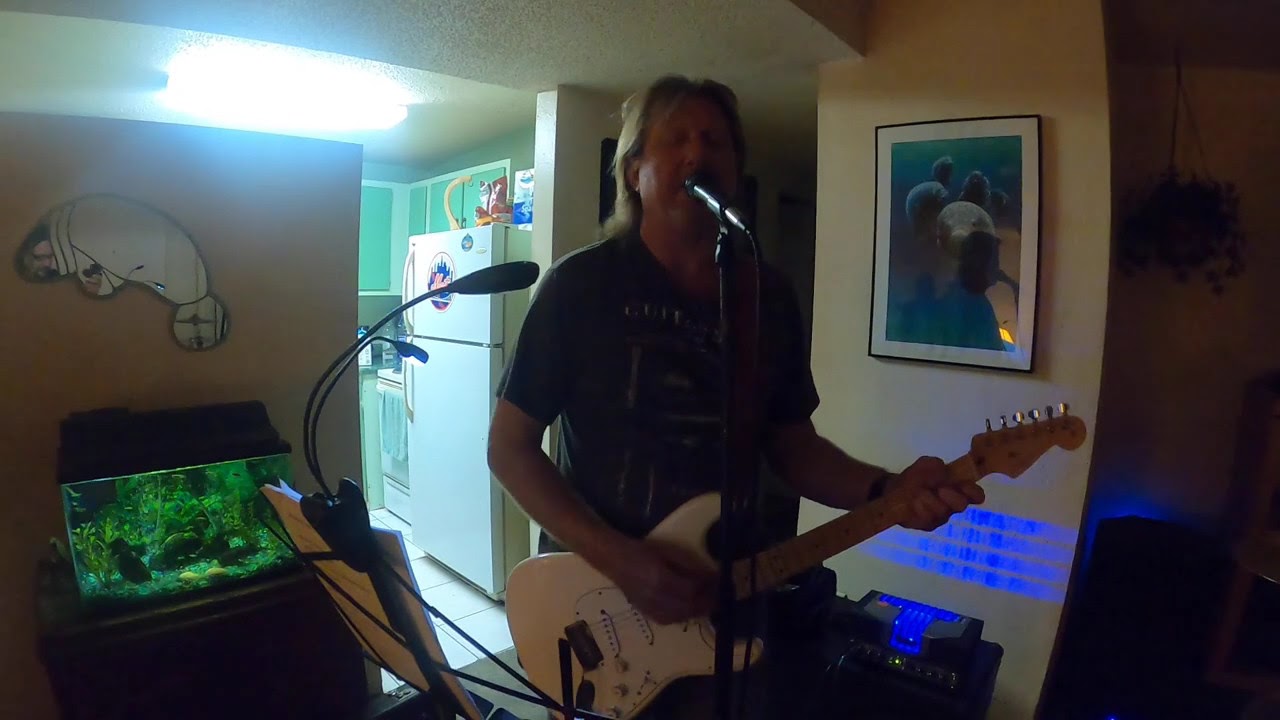The detailed image shows a person standing in their home, centered in the foreground, passionately playing a white electric guitar with a light brown neck while singing into a black microphone on a stand. The person, who appears male and has light skin, is dressed in a gray t-shirt adorned with a black and white design. Both of his hands are engaged with the guitar; the left on the neck and the right on the strings. 

Adjacent to him on the right is a music stand, clipped with a table lamp and several sheets of white paper. To his left is an aquarium perched on a side table, filled with various green vegetation and housing a few visible fish. Above the aquarium, a mirror shaped like a manatee is mounted on the wall. The room has a cozy atmosphere with a cream-colored ceiling, featuring a bright white light in the adjoining kitchen, visible in the background. The kitchen contains a white refrigerator and a white oven. Additionally, the room's decor includes several paintings and posters, contributing to a personalized and artistic environment.